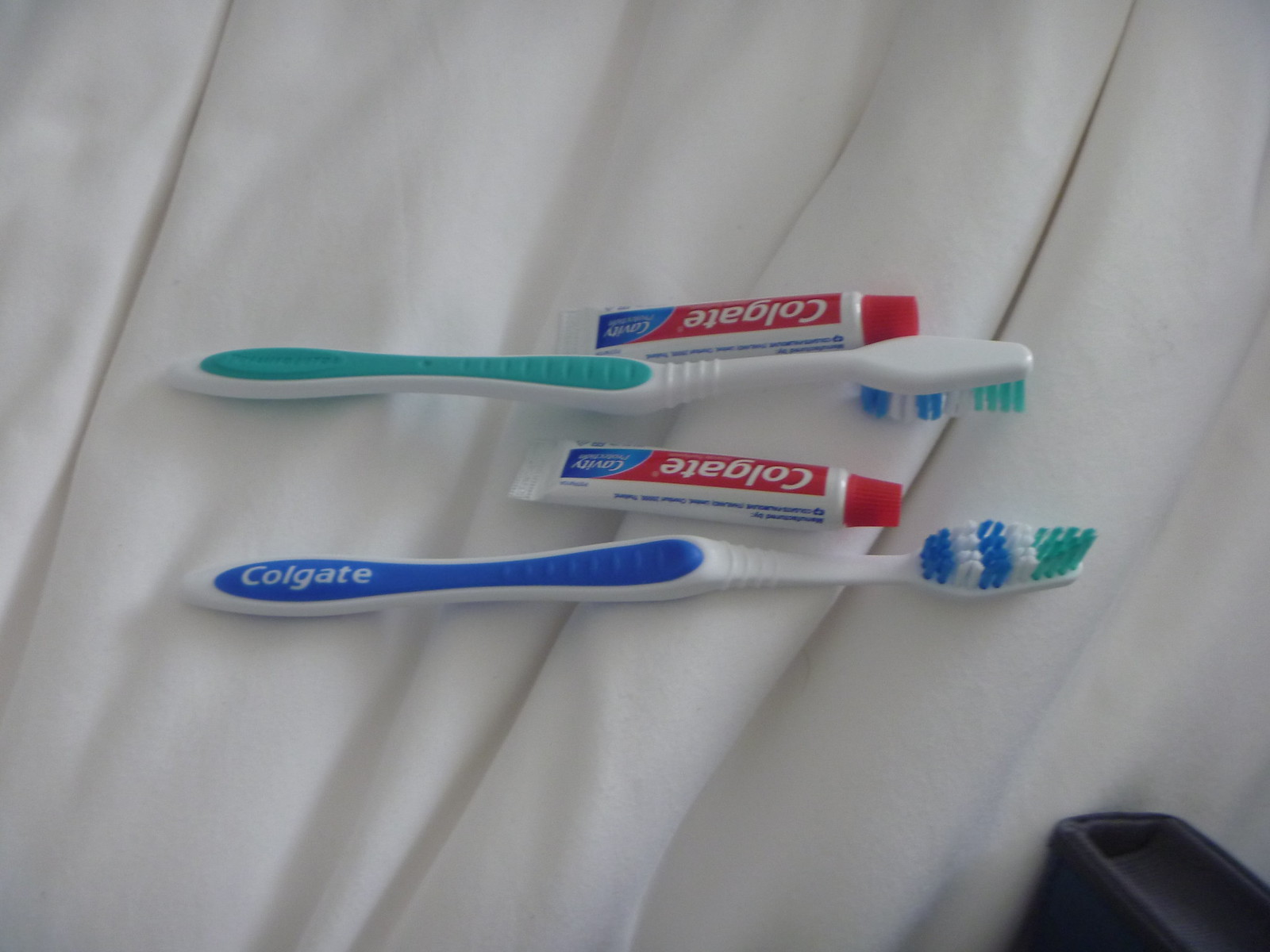This photograph depicts two toothbrushes and two small travel-sized tubes of Colgate toothpaste arranged on a pure white, slightly bunched-up fabric that resembles a blanket or sheet. The toothbrushes are positioned horizontally, one with its bristles facing up and the other with its bristles facing down. The toothbrush with its bristles up has a white handle with a blue grip, labeled "Colgate," and its bristles are a combination of blue, white, and turquoise. The toothbrush with its bristles down features a white handle with a turquoise grip, and similar multi-colored bristles. Each toothbrush is paired with a small tube of Colgate toothpaste, identifiable by their white tubes with red caps and red labels that read "Colgate." Additionally, there is a faintly visible, black, curved object in the bottom right corner of the image.